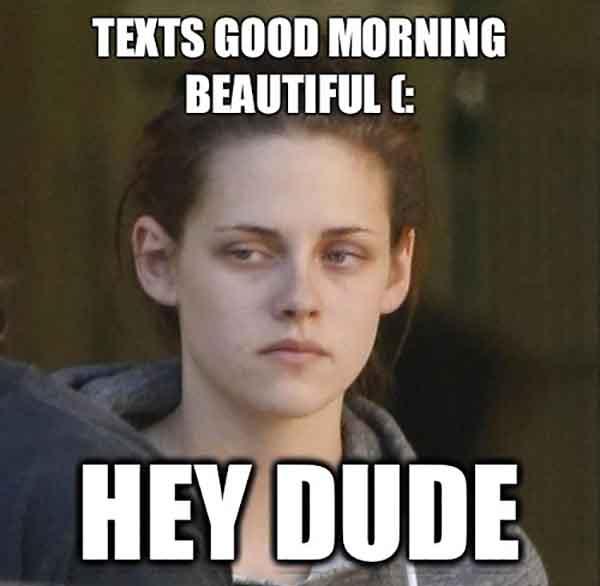The meme features a centered image of actress Kristen Stewart, who has pale skin and brown hair pulled back, dressed in a gray hooded sweatshirt. Her expression is neutral, with her mouth closed, looking slightly to the left of the camera. The top of the image displays the text "GOOD MORNING BEAUTIFUL" in bold, all-capital white letters with a black outline, accompanied by a smiley face. At the bottom, the text "HEY DUDE" is written in even larger bold, all-capital white letters with a black outline. In the bottom left corner, in front of Kristen Stewart but partially obscured by the text, there is the visible shoulder of another person wearing a dark gray sweatshirt. The background is out-of-focus, presenting a blurred mix of green and brown hues, likely indicating an outdoor or natural setting, though indistinct and unclear.